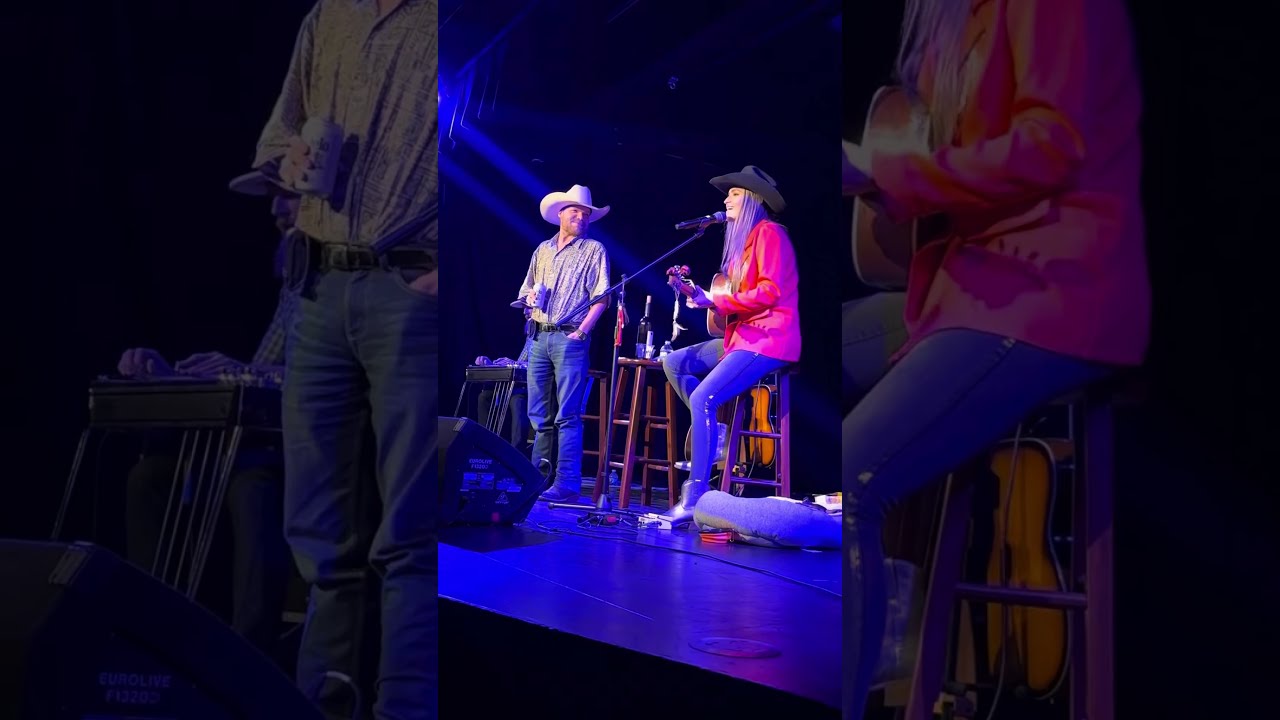In this portrait-mode image, we see a live country music performance featuring a man and a woman on a somewhat dimly lit, blue-hued wooden stage. On the left stands a man clad in blue jeans and a long-sleeve flannel shirt with its sleeves rolled up to his elbows. He wears a white cowboy hat and holds a microphone while looking to the right at his partner, who is seated. The man also appears to be holding a can and has his other hand in his pocket.

The woman seated on a simple wooden barstool is the focus of the stage. She dons a tight pair of blue jeans, black short boots, a black cowboy hat, and a red long-sleeve shirt over which she wears a pink blazer. She is playing an acoustic guitar and singing into a black microphone that is mounted on a stand leaning towards her. Beside her is another wooden barstool that holds several drinks and other items. The stage is bathed in blue light, adding to the intimate ambiance of the performance. Despite the clutter on the floor beside the woman, the essence of live country music is vividly captured in this atmospheric scene.